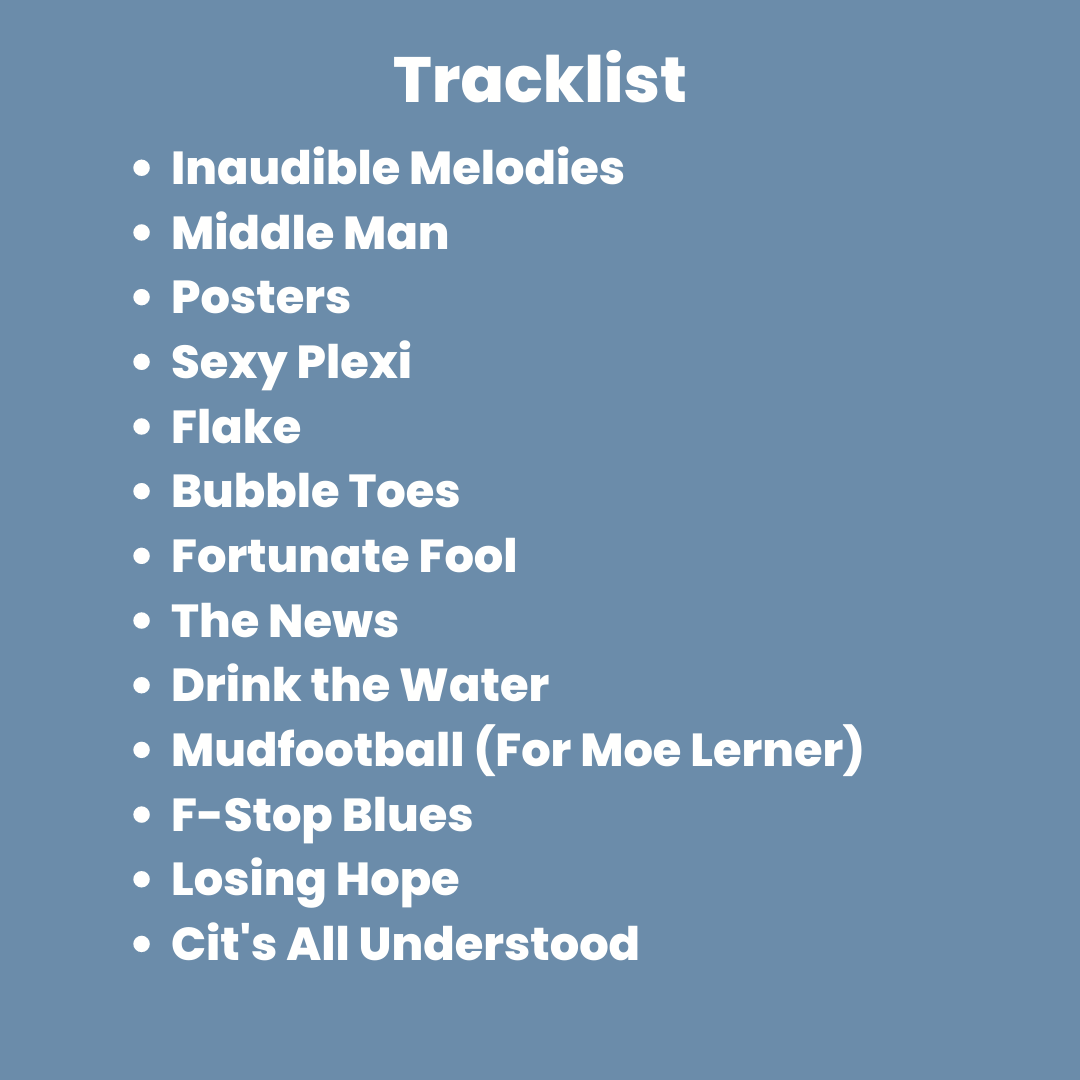The image showcases a blue background with a prominently displayed, bold white title in the center at the top, reading "Track List" in an official, Helvetica-like font. Below the title, a detailed list of bullet points—also in white text—includes the following items: Inaudible Melodies, Middle Man, Posters, Sexy Plexi, Flake, Bubble Toes, Fortunate Fool, The News, Drink the Water, Mud Football (with "for mole learner" noted in parentheses), F-Stop Blues, Losing Hope, and Shit’s All Understood. The clean and minimalistic design focuses solely on the text, providing a comprehensive tracklist in a straightforward layout.